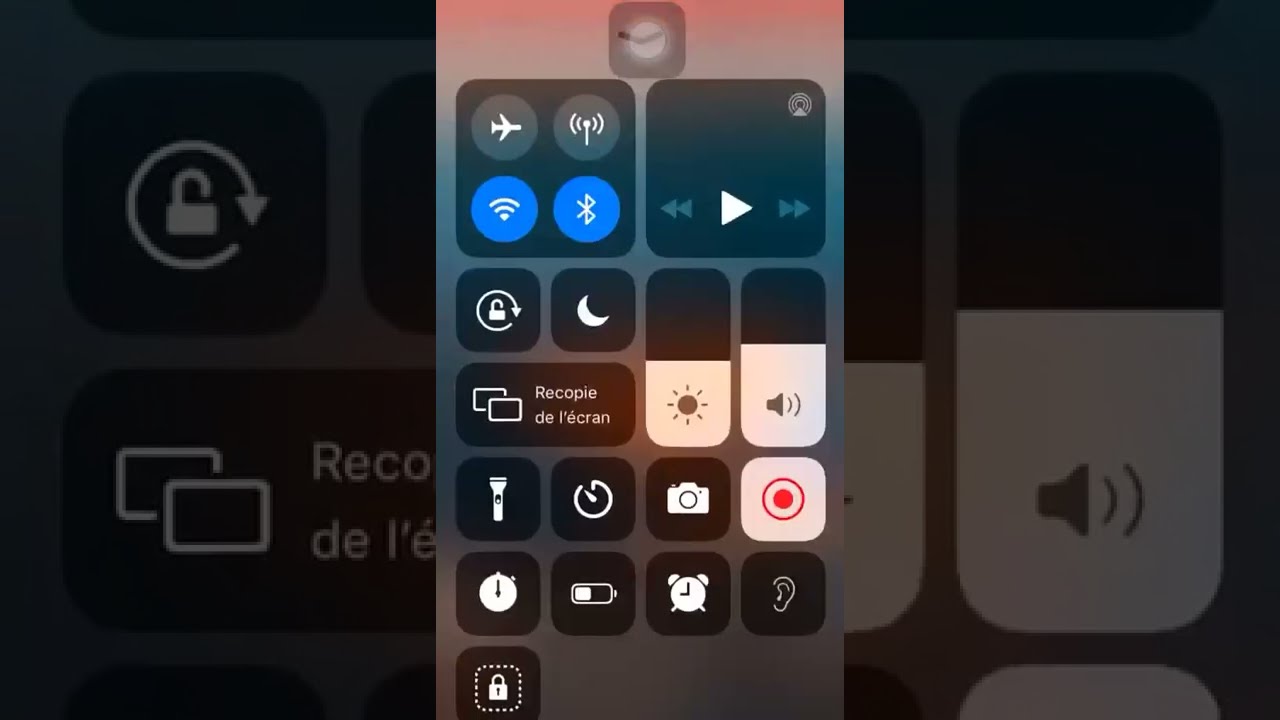This is a detailed screenshot of an iPhone's Control Center, captured via screen recording, which is indicated by the illuminated red screen record button. The image primarily features the Control Center that appears when swiping down from the top-right corner of the screen. It shows a variety of control toggle icons within black squares, such as airplane mode, Wi-Fi, Bluetooth, flashlight, mobile data, screen rotation lock, Do Not Disturb mode, and a timer. The icons for Wi-Fi and Bluetooth are highlighted in blue, indicating they are active. The layout has a gray-to-pink gradient background. Notably, the screen mirroring icon is labeled in French as "Recopie de l'écran." Additionally, the left and right edges of the image present a zoomed-in, darkened version of the same Control Center, serving as a decorative border.